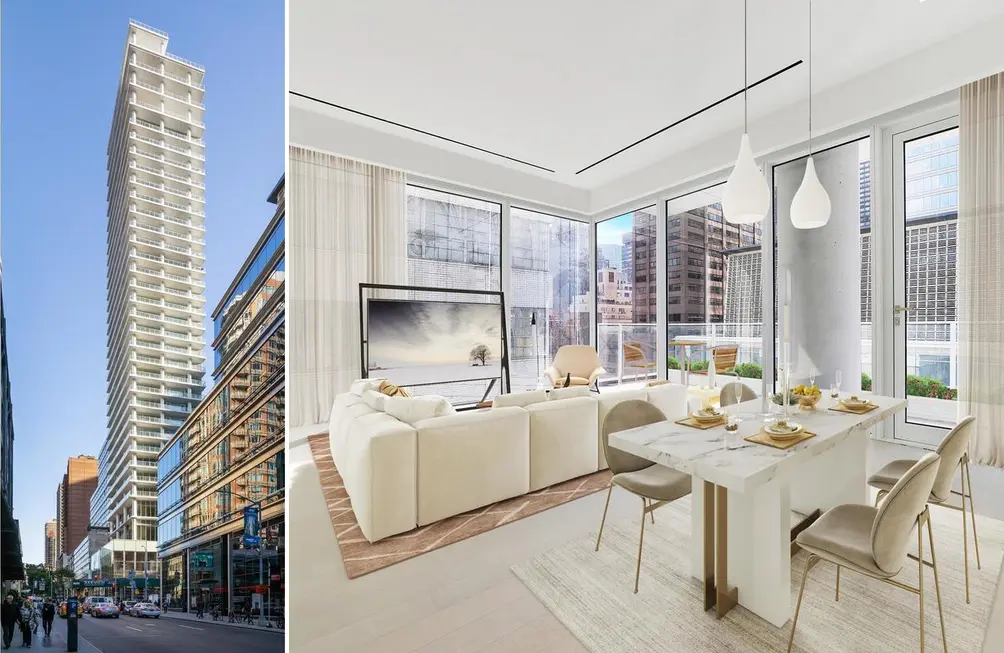**Caption:**

*Image 1: A bustling cityscape captures the vibrancy of urban life. Towering skyscrapers dominate the skyline while cars navigate the busy streets below. Pedestrians can be seen strolling along the sidewalks past various storefronts, their signs prominently displayed. The interplay of light and shadows adds depth to the scene, suggesting it is late afternoon, an hour before dusk. The medium blue sky hints at the day's transition into evening.*

*Image 2: Inside a cozy, modern home with glass walls adorned with white curtains, offering a stunning view of downtown's central buildings. The living space features two wall-mounted lights, a beige couch placed on a red rug, and a flat-screen TV on a stand reminiscent of a chalkboard. In the corner, a table with four chairs is arranged, completing the inviting, urban retreat.*